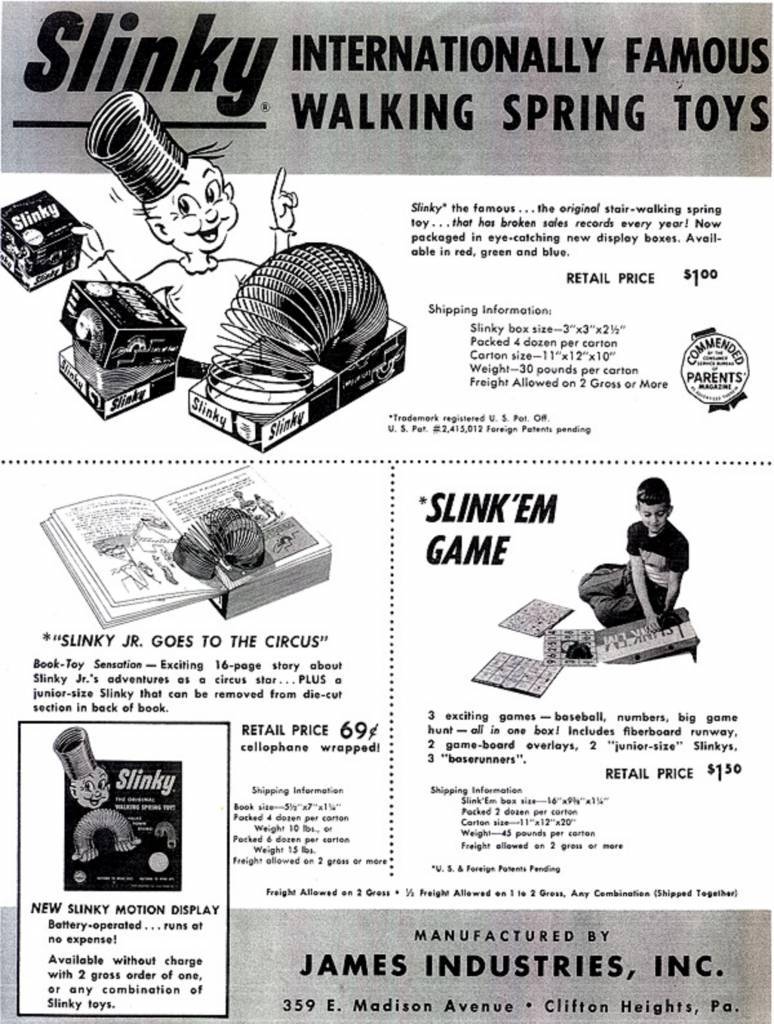The black and white, halftone-style advertisement for the famous Slinky toy presents a nostalgic look, reminiscent of old comic books or newspaper ads. At the top, bold text reads, "Slinky, Internationally Famous Walking Spring Toys," highlighting the toy's global acclaim. The center illustration features a cheerful cartoon boy with a Slinky perched on his head while holding a Slinky box in one hand and pointing upward with the other. Below him are two Slinkys: one partially visible inside a box, the other stretched out between the opened halves of a flattened box. Promotional text boasts, "Slinky, the famous, the original stair-walking spring toy," and notes its consistent record-breaking sales. The toy is now available in eye-catching red, green, and blue display boxes, each retailing for $1.

To the left, a smaller section advertises "Slinky Jr. Goes to the Circus," an exciting 16-page storybook featuring Slinky's adventures as a circus star. Just below is an ad for the "Slinkum Game," a ramp game involving the Slinky, priced at $1.50, where a young boy is depicted playing with it.

At the bottom of the ad, in a gray bar, the manufacturer information reads, "James Industries Inc., 359 East Madison Avenue, Clifton Heights, Pennsylvania," ensuring eager customers know where this beloved toy originates.